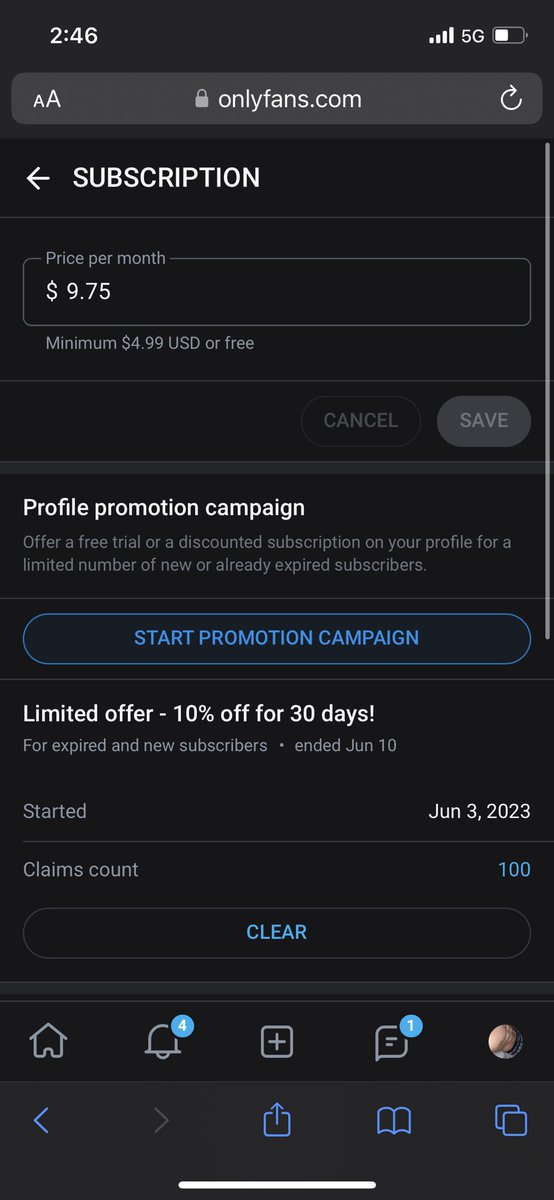In the image of an iPhone, the device is clearly connected to a strong 5G network with a battery life at 50%. The time displayed on the screen is 2:46. On the browser, the URL in the search bar reads "onlyfans.com". 

At the top left, there is an "AA" icon, and on the top right, there is a circular arrow icon. Below the URL, the word "SUBSCRIPTION" is written in white, all caps. The subscription price is listed as $9.75 per month, with a note that a maximum of $4.99 in U.S. dollars is free. There are two buttons: a 'Cancel' button and a 'Save' button, the latter being illuminated.

Further down the screen, it mentions "Profile Promotion Campaign" offering a free trial. A highlighted blue box with blue text indicates that you can start your promotion campaign. The promotion is a limited offer of 10% off for 30 days, starting on June 3rd, 2023. It shows that the claims count is at 100, with a "Clear" option in blue.

At the bottom of the screen are various icons. The alert icon has four notifications marked by a blue box, and the messages icon has one notification. Most of the icons appear semi-transparent, except for a personalized icon on the upper right row, which has a yellowish-tan color.